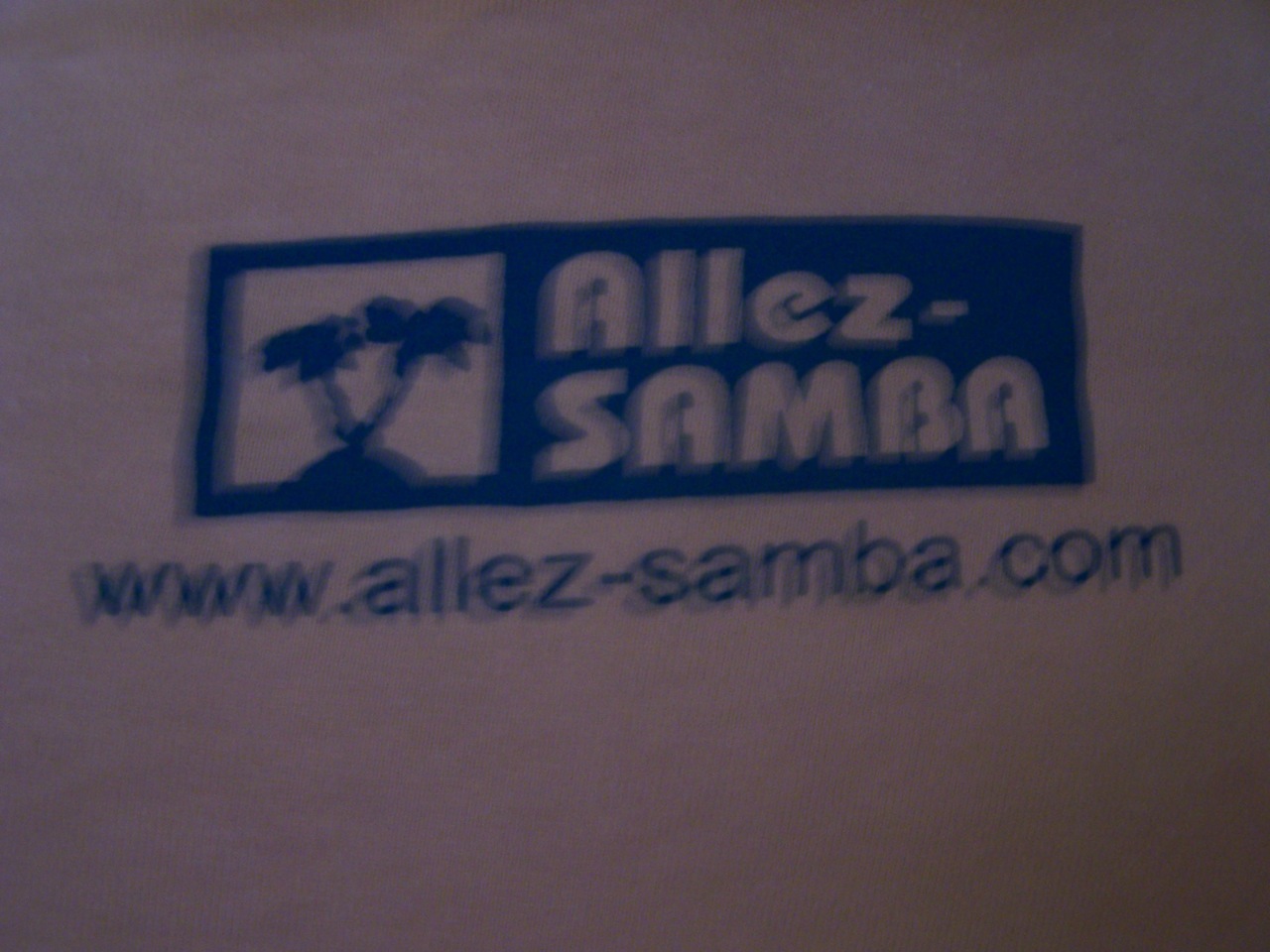The image features a slightly blurred logo set against a white background, resembling a sign or a piece of paper. The focal point is a rectangular, landscape-oriented logo with a blue background. On the left side of the rectangle is a white square containing a simple, block-style illustration of two blue palm trees. This square takes up approximately one-third of the logo. The right side, which occupies the remaining two-thirds of the rectangle, displays the brand name "ALLE-SAMBA" in a curvy, elegant font.

Below the blue rectangle, a website address exceeds the logo's width in blue letters, reading www.alle-samba.com. The entire logo, including the website address, occupies about one-third of the image's total white space. The image itself is slightly out of focus, drawing attention to the design and text despite the blur.